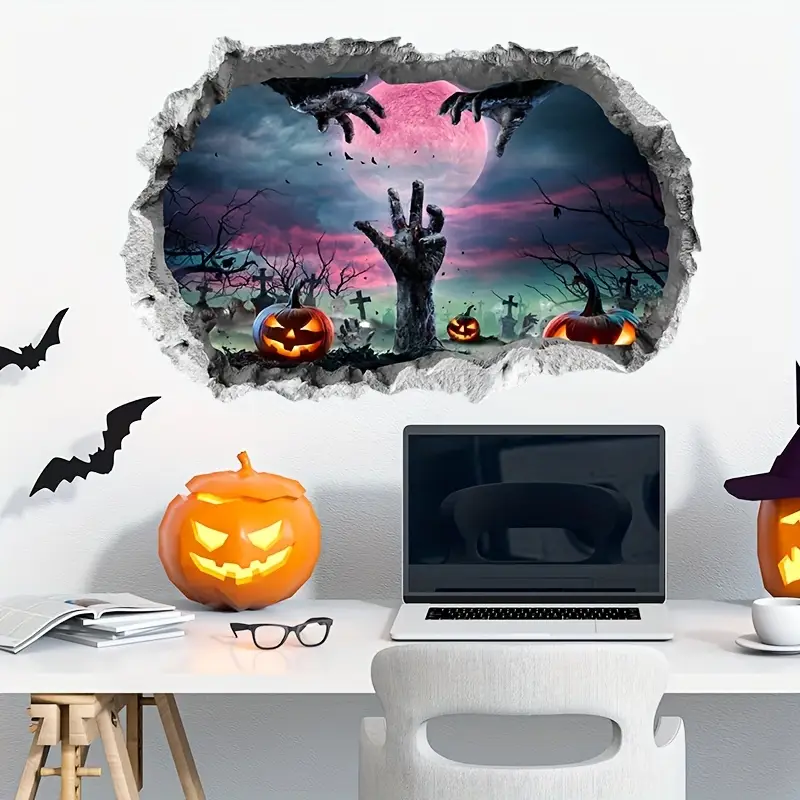In the image, we see a white computer table supporting an open white laptop with black keys. A white chair is immediately in the foreground. On the table, to the left of the laptop, there's a pair of glasses next to a pumpkin with its top slightly removed. To the right, there's another pumpkin partially visible, adorned with a black witch hat, and a white cup sits on a plate. A stack of books with the top one open is also to the left, and two black bats hang on the left wall edge. Below the table, a wooden holder is visible. The background shows a white wall with a rough, broken hole, through which a spooky Halloween scene is visible: dark, glowing pumpkins with zombie heads and hands emerging from the ground, crosses, tombstones, and a purplish-pink moon illuminating the eerie sky. The overall setting exudes a Halloween vibe with its array of ominous decorations.